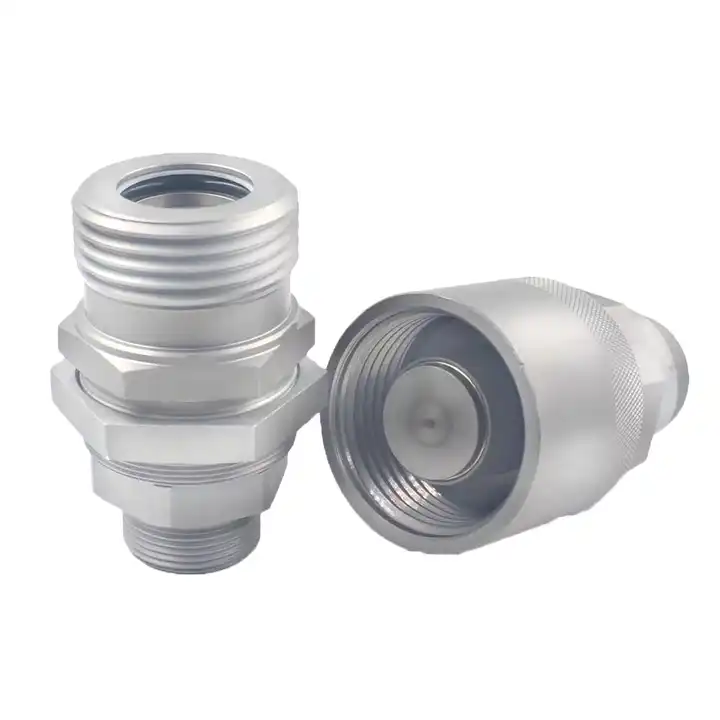This image features a highly detailed, computer-generated rendering of two industrial tool pieces, presented on a pristine white backdrop. To the left, standing upright, is a silver-gray washer with precisely crafted grooves around its head, suggesting it can securely fit into the threaded lock positioned to its right. The washer’s reflective, smooth surface and perfect geometric form give it a digitally rendered appearance, yet accurately model a real washer. The threaded lock, also appearing in silver-gray, is lying on its side, revealing its hollow, threaded interior and dome-shaped top. Both objects exhibit an impeccable finish, with no imperfections, reinforcing the notion of a CGI render intended to mimic the exact specifications of actual hardware components.